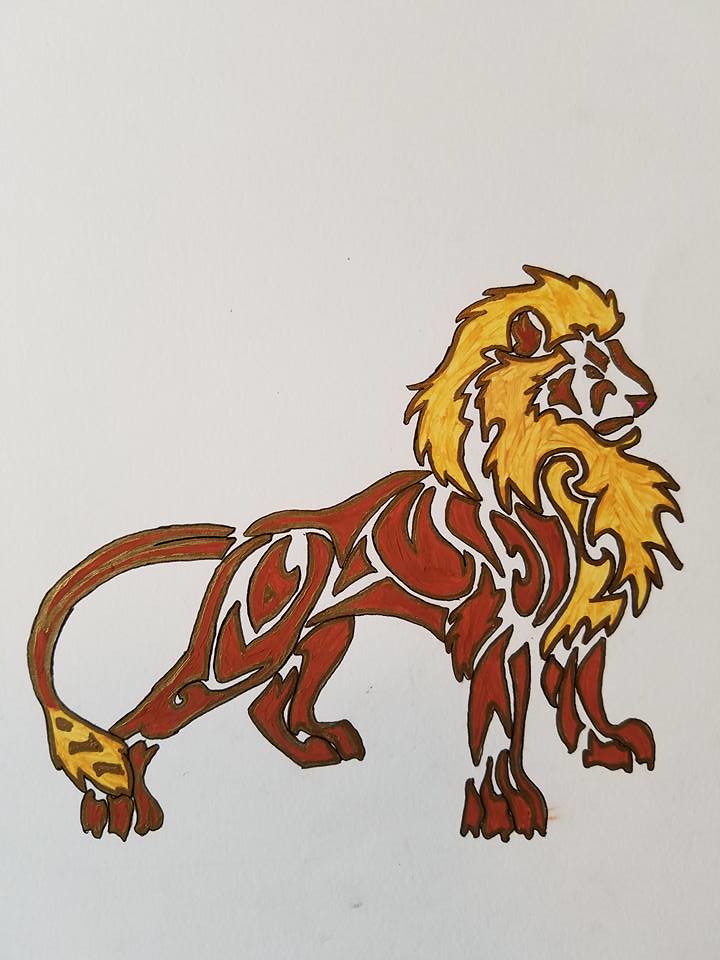In this image, a hand-drawn sketch of a male lion stands out against a light gray background. The lion is oriented to face the right side of the image, showcasing a detailed side profile. Outlined in fine black marker, the body is filled with fragmented shapes and colored predominantly in dark brown, with some areas appearing slightly lighter, possibly suggesting an uneven coloring process. The lion's mane, which flows from the top of its head down the sides and under its chin, is shaded in yellow or light gold. Its face is predominantly white with brown highlights and a reddish nose. The tail, curving back towards the center, is dark red, with the tip colored yellow featuring a series of brown stripes or spots. This sketch exudes a sense of pride and majesty, emphasized by the lion's proud stance, perked ears, and upright chest.